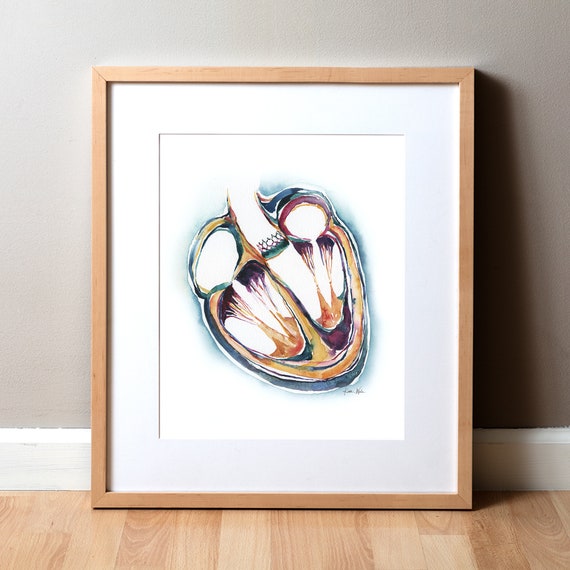This indoor photo showcases a piece of art propped against a wall. The artwork is encased in a narrow, light wooden frame and leans against a soft grey wall with white baseboard trim and what appears to be a laminate wood floor. The framed piece presents an intricate drawing of a human heart, detailed with the left and right chambers and a stent opening to a valve. The heart's interior is vividly colored with muted blues, deep reds, and wine tones. Although the heart shape and anatomical details are clear, some may interpret the image as abstract or reminiscent of a cutaway view of some organic form, like a seed or berry, due to its compartmentalized appearance. The overall scene is illuminated gently from above, emphasizing the artistic and introspective nature of the piece.